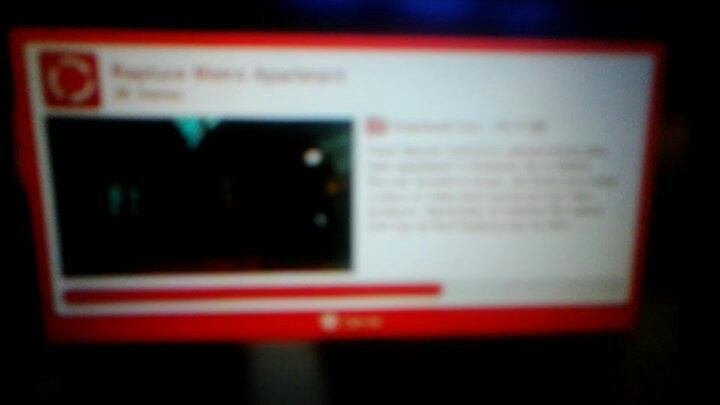The image depicts a highly blurry text-filled card or sign framed within a thin red rectangular border. The background of the entire scene is dark, with hues of black and bluish reflections creating a dim ambiance, possibly suggesting a dark room. At the top left corner of the bordered card, there is a distinct red square logo featuring a white circle inside, accompanied by an adjacent red headline text, all blurred beyond recognition. The main portion of the card's interior is white, housing a rectangular picture on the left side, which itself appears indistinct and suffused with dark tones and some blue illumination, while the text on the right seems to describe the image. A red line, reminiscent of a progress bar such as seen in video games, is positioned at the bottom, with a partial, indistinct white logo centered within the red border beneath it. The overall texture and details of the text are so obscured that the intended content remains unreadable, conveying an overall sense of mystery and vagueness.